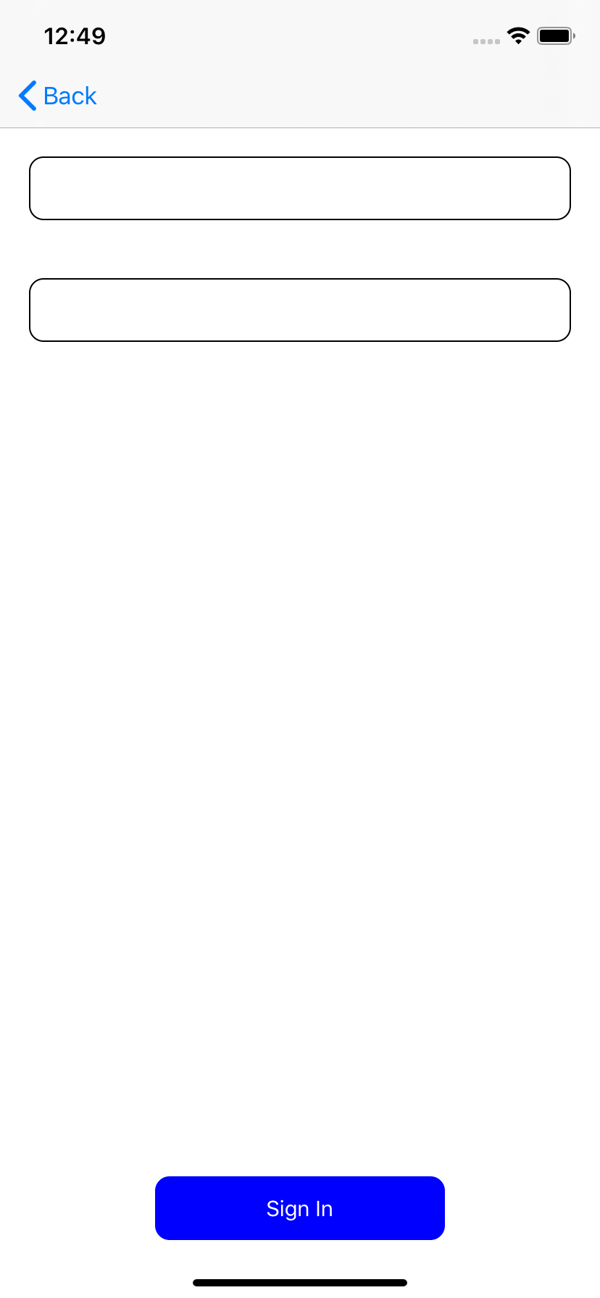The image displays an iPhone interface screen showcasing a typical login page design. At the top-left corner, the time is indicated as "12:49," and on the top-right corner, several status icons are visible: a series of four grey dots, the WiFi symbol, and a fully charged battery icon. Below the status bar on the left, the word "Back" is displayed in blue text with an accompanying left-pointing arrow. This section has a grey background which contrasts with the white background below it.

Further down, two empty text fields with subtle black borders stretch horizontally from edge to edge against the white background. Below these fields, the remaining white space extends until the bottom of the page, where a prominent blue rectangular button with rounded corners is centered. The button features "Sign In" written in white text. Just beneath this button, a small notch, resembling a black line, is visible.